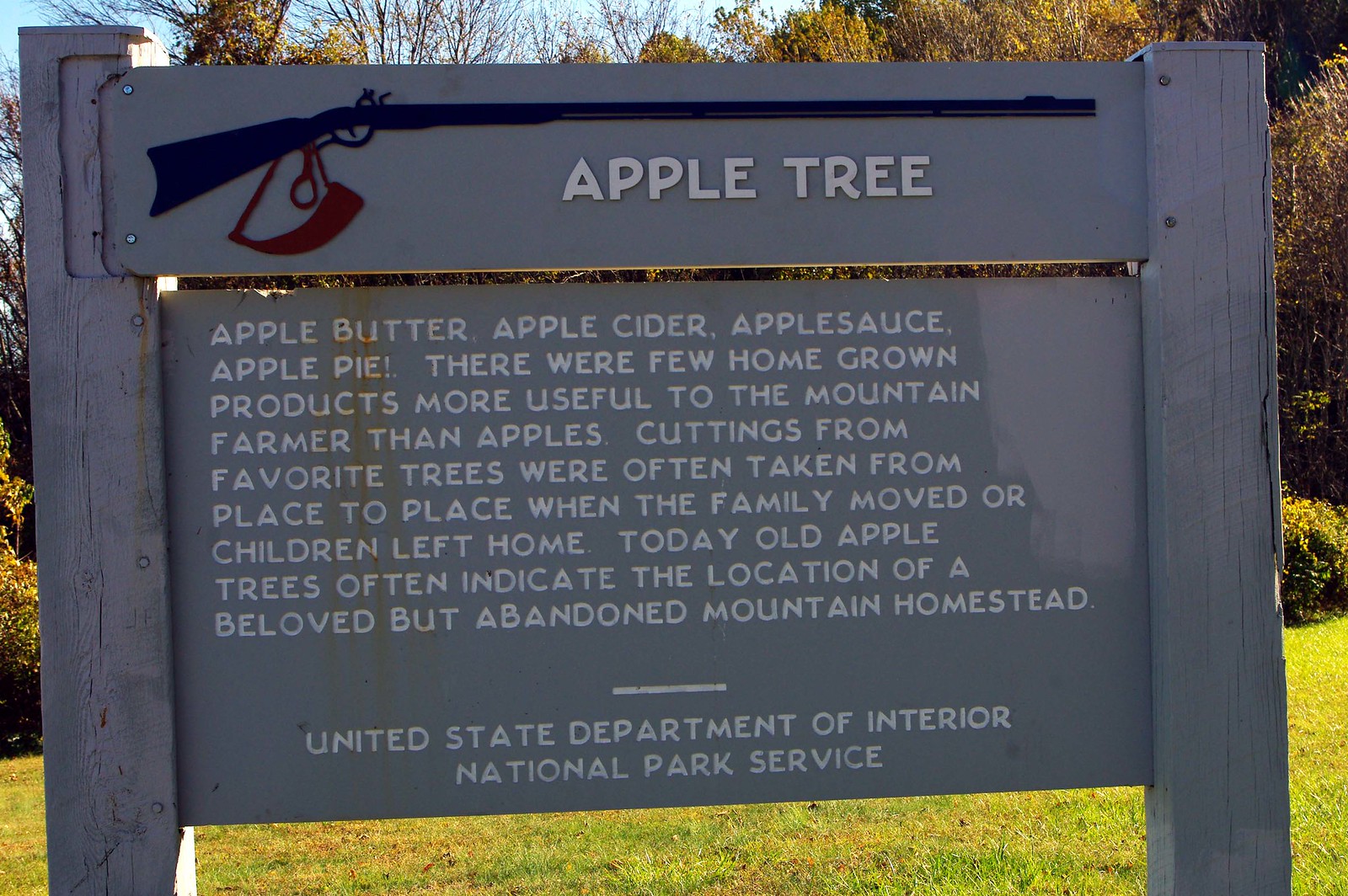This image depicts an outdoor wooden sign, likely situated in a public park or green space. The sign itself is painted green and prominently features an outline of an old-style rifle, beneath which it reads "Apple Tree" in white font. Below this, the sign lists several apple-related items: "Apple Butter, Apple Cider, Applesauce, Apple Pie." The sign narrates: "There were few homegrown products more useful to the mountain farmer than apples. Cuttings from favorite trees were often taken from place to place when the family moved or children left home. Today, old apple trees often indicate the location of a beloved but abandoned mountain homestead." At the bottom of the sign, following a small horizontal white line, it states: "United States Department of the Interior National Park Service." The background of the image includes some grass, further suggesting the sign's placement in a natural, park-like environment.